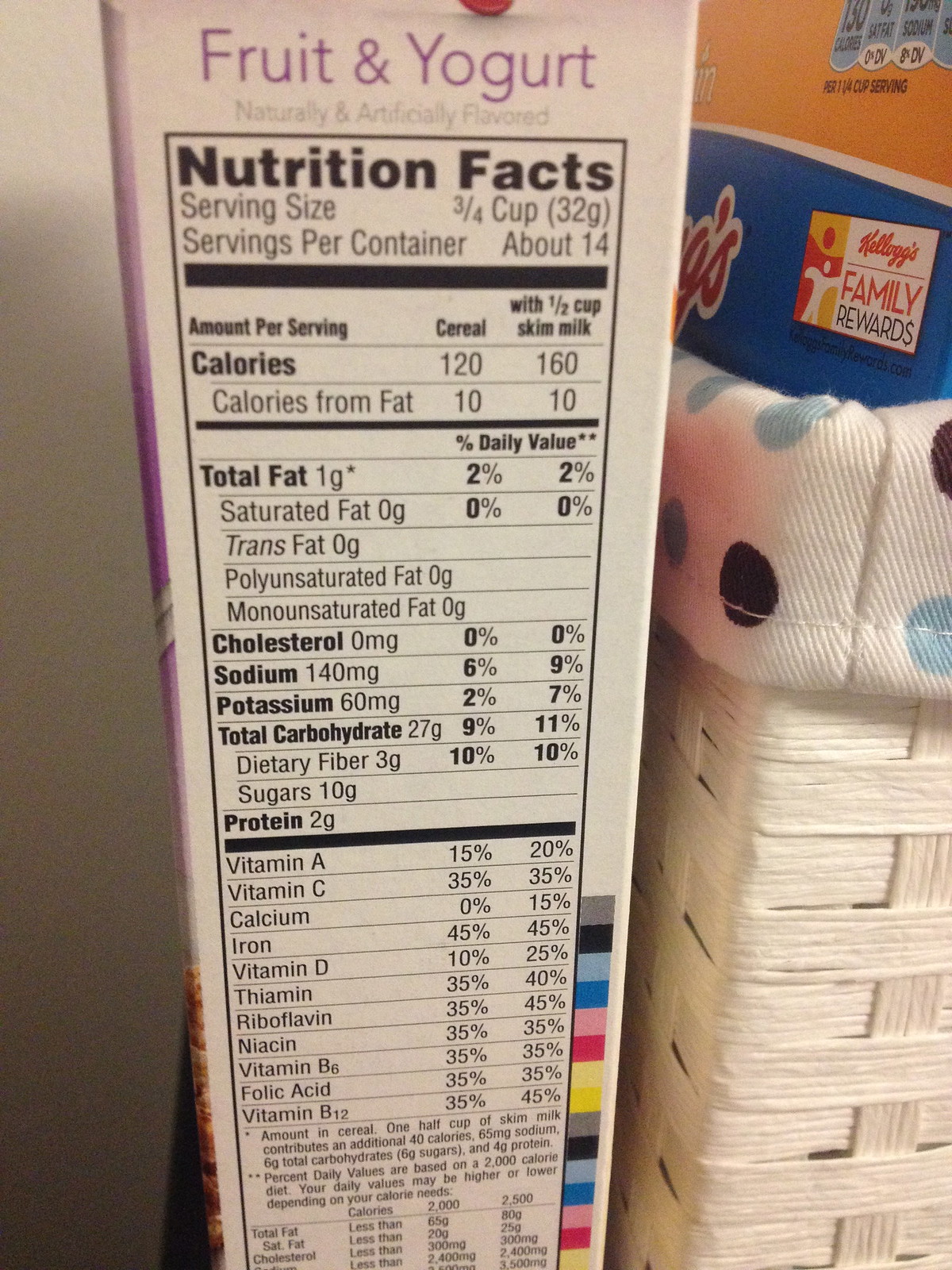The photograph, taken indoors in color and portrait mode, features the vertical side of a narrow food box against a white background. The top edge of the box displays "Fruit and Yogurt" in purple text followed by "Naturally and Artificially Flavored" in gray. Below this, a long, narrow "Nutrition Facts" label is visible, indicating a serving size of three-quarters of a cup. The label includes detailed nutritional information: 10 calories from fat, 1 gram of total fat with 0 grams of trans and saturated fats, zero cholesterol, 140 milligrams of sodium, 60 milligrams of potassium, 27 grams of total carbohydrates, 3 grams of dietary fiber, 10 grams of sugars, and 2 grams of protein. Adjacent to the box, a white wicker basket with a folded white cloth lining adorned with dark blue and light blue polka dots partially holds another box, presumably of cereal. The words and layout strongly suggest the product may be a Special K Fruit and Yogurt cereal variant.